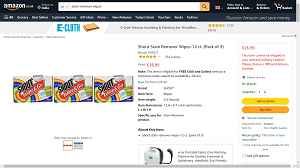This is a pixelated screenshot of a webpage from Amazon.co.uk, viewed at a distance. The image is not very clear, but discernible details indicate that the user is accessing their account and browsing items in their shopping basket. The user appears to be looking for a 12-pack product, possibly kitchen rolls, toilet rolls, tissue packs, or wipes, priced at approximately €25.99. Notably, the item is indicated as in stock by green text, though red text also appears, which may suggest pre-order status or another condition. The screenshot has a white bottom edge, indicating it might have been superimposed onto a white background. Further details include dimensions and additional composition information about the item for sale.